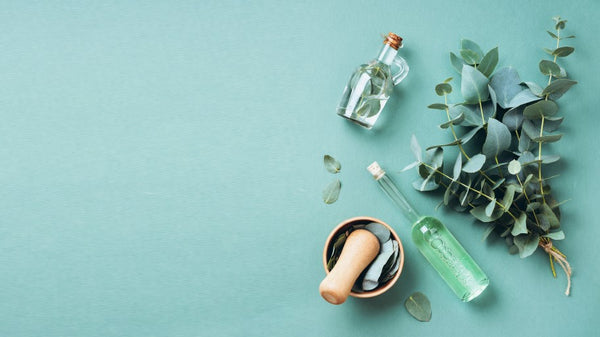The image showcases a collection of objects on a Tiffany box-colored bluish-green background, predominantly on the right side. Central to the arrangement is a set of botanical elements and tools. 

From a bird's eye view, a bottle with a long, thin neck and a clear light-colored cork is situated towards the bottom. This bottle contains a light green liquid. Above this is a cluster of stems adorned with small, pointed green leaves, tied at the base with a burlap-like string.

Positioned further up, there is a shorter bottle featuring a handle and topped with a goldish-brown cork. This bottle contains a clear liquid with several leaves immersed inside. To the left of the stems is a wooden mortar and pestle, with the mortar holding additional leaves.

Scattered around the objects, there are a few loose leaves – three specifically between the smaller bottle and the mortar, with one leaf lying between the mortar and the taller bottle. Overall, the setup suggests a natural, possibly herbal theme with ingredients and tools for leaf extraction on a serene bluish-green backdrop.